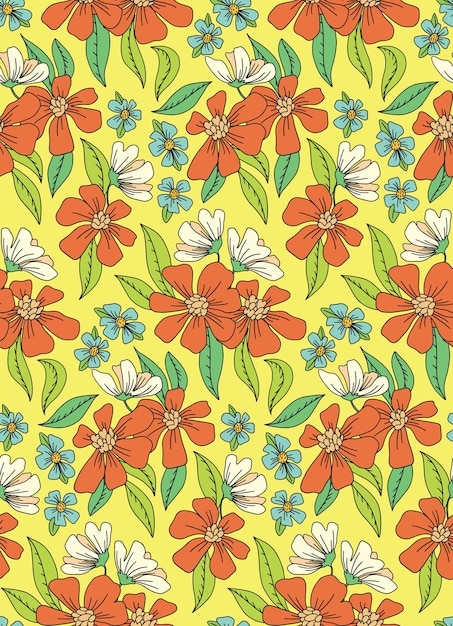The image is a horizontally rectangular, multi-colored illustration of various flowers with a simple, pale yellow background and no borders. Dominating the composition are vibrant red-orange flowers, the largest and most prominent, some of which contain small, round berries-like elements. Scattered among these are medium-sized white flowers shown mostly in side profile, making them appear less prominent. The smallest blue flowers are interspersed throughout, filling the spaces between the other blooms and adding decorative touches. Additionally, there are occasional orange flowers present. The leaves exhibit varying shades of green, ranging from pale to dark hues with a slight bluish tint. Some leaves show detailed striations and hatch marks, contributing subtle texture to the overall artwork. The arrangement of the flowers appears random and lacks a specific pattern.